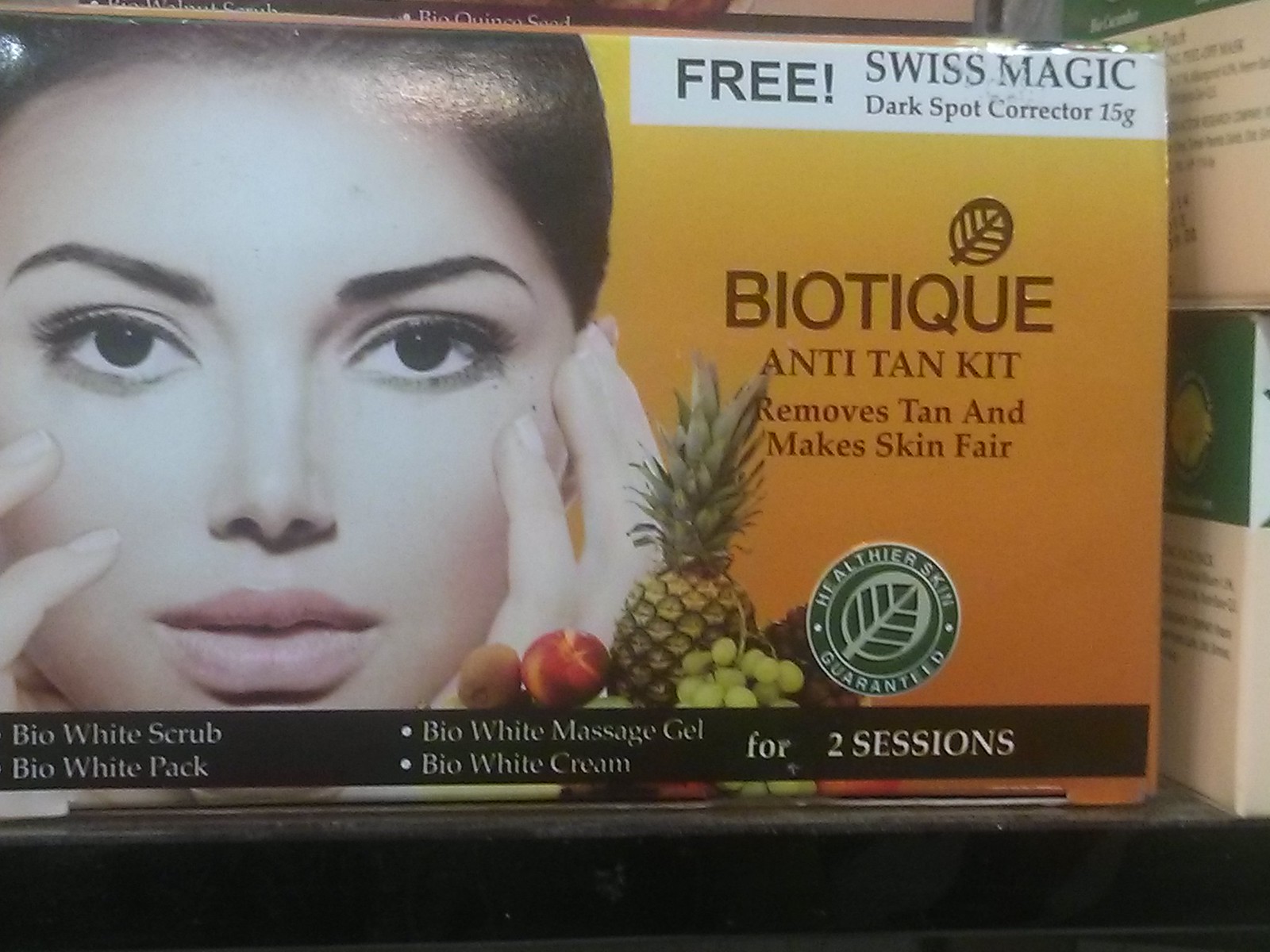The image is a street or store advertisement for a facial care product aimed at skin brightening and tan removal. It features a close-up of a beautiful Asian woman with dark hair, heavy makeup, including black eyebrows and eye makeup, and a look of contemplation with her hands gently framing her face. On the top right of the advertisement, set against a bright orange background, are bold white and black letters stating, "Free Swiss Magic Dark Spot Corrector 15g." Adjacent to this, in brown letters on the orange section, are the words, "Biotic Anti-Tan Kit - Removes Tan and Makes Skin Fair." Below this text, there are illustrations of various fruits such as pineapples, peaches, and grapes, likely highlighting natural ingredients. Additional product descriptions include "Bio White Scrub," "Bio White Pack," "Bio White Massage Gel," and "Bio White Cream for Two Sessions," all detailed in a green and white circle at the bottom. The image quality is somewhat faded, and the overall look of the advertisement is cluttered and slightly dirty.